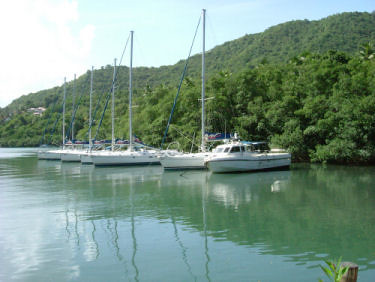In this vibrant image, we observe a serene waterfront scene featuring a line of six boats, predominantly white with occasional black or blue stripes, anchored near the shore. The boats, some of which appear to be sailboats with their grey masts standing tall, are positioned in the middle of the frame, creating a picturesque alignment that extends from the center to the far right. The vessel furthest to the right lacks a mast and showcases a curved front with windows. 

The tranquil water reflects the lush greenery of the surrounding landscape and the bright blue sky peppered with white clouds in the top left corner. The upper half of the photo showcases an expansive, forested hill or small mountain carpeted with dense trees and vegetation, accentuating the natural beauty of the background. Additional bushes and trees align the waterfront, enhancing the scenic and peaceful setting.

In the bottom right corner, a green leaf and a post hint at the presence of a dock, although the dock itself is not directly visible. The clear, sunny day bathes the scene in vibrant light, creating a peaceful and inviting atmosphere.